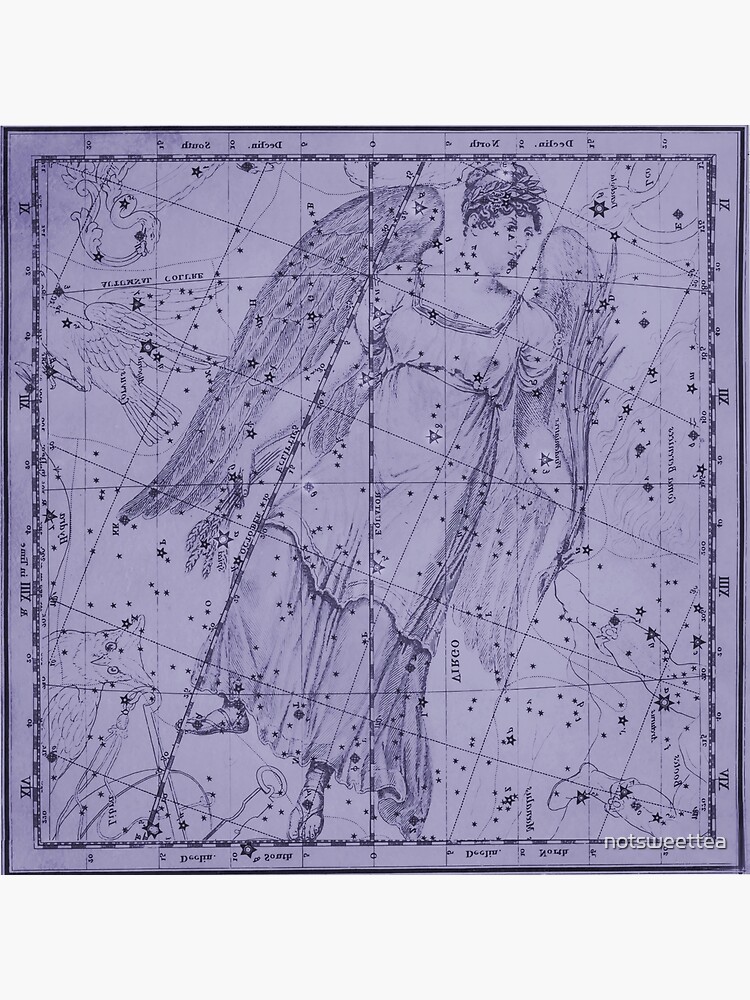The image depicts a meticulously sketched diagram with a light gray background, showcasing an intricate map of stars and constellations peppered with small black dots. At the heart of the chart, drawn in a dark gray pencil-like style, is a female angel in a slight white gown, reminiscent of 1800s attire. She stands diagonally at the center, adorned with extensive wings and a wreath in her hair, and holds another wreath in her hand. Thin-strapped sandals adorn her feet. Surrounding the angel are additional detailed drawings, including depictions of a snake, a bird, and an owl, alongside various legs and other constellation shapes. The chart is bordered by small foreign text and Roman numerals running vertically along its sides.